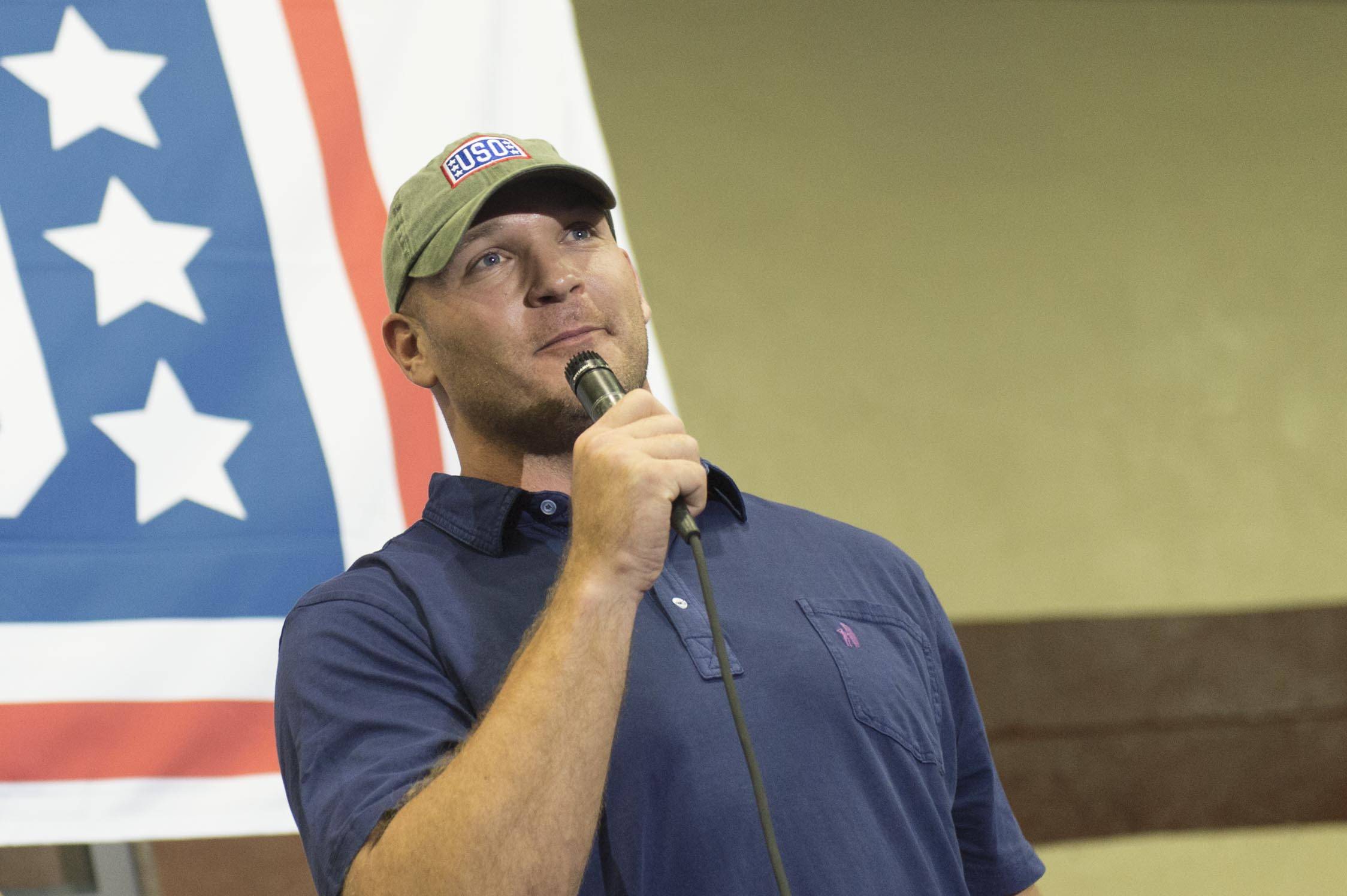In the image, a man is captured mid-speech, holding a black microphone with a black wire in his right hand close to his mouth. He has light-colored eyes and is wearing a blue polo t-shirt. His head is adorned with a yellowish-gray cap featuring the text "USO" written in white within a blue rectangular background. The man is slightly leaning to the left and appears to be smiling.

The backdrop includes a diagonally framed light brownish-yellow wall with a dark chocolate brown border running from his bicep area to the right of the image. On the left side, there's a partially visible large flag with red lines and blue sections adorned with white stars, indicating a patriotic setting.